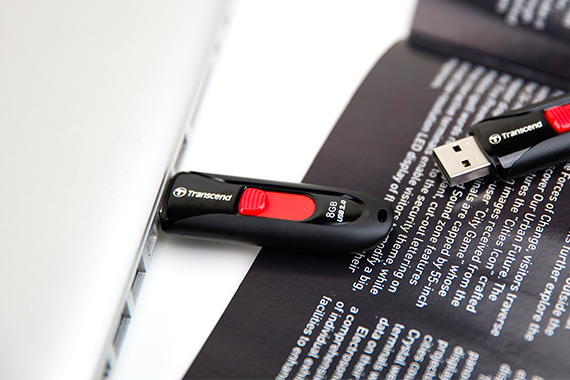The indoor photograph, styled in landscape orientation, captures two nearly identical flash drives, both black with red accents. One flash drive, labeled "Transcend 8GB USB 2.0," is plugged into the side of a sleek, silvery-white laptop on the left-hand side of the image. The other flash drive, which bears the same "Transcend" branding and red knob, is positioned to the right, resting on top of a black book or magazine with white text. This text is partially readable with phrases like "Forces of Change" and "Visitors Traverse Discover Our Urban Future," but much of it is out of focus. The magazine is angled from the bottom left to the top right, creating a dynamic backdrop. The plugged-in flash drive casts a shadow over the book's edge, while the unplugged drive casts a slight reflection on the black paper. The entire scene is set against a white background.